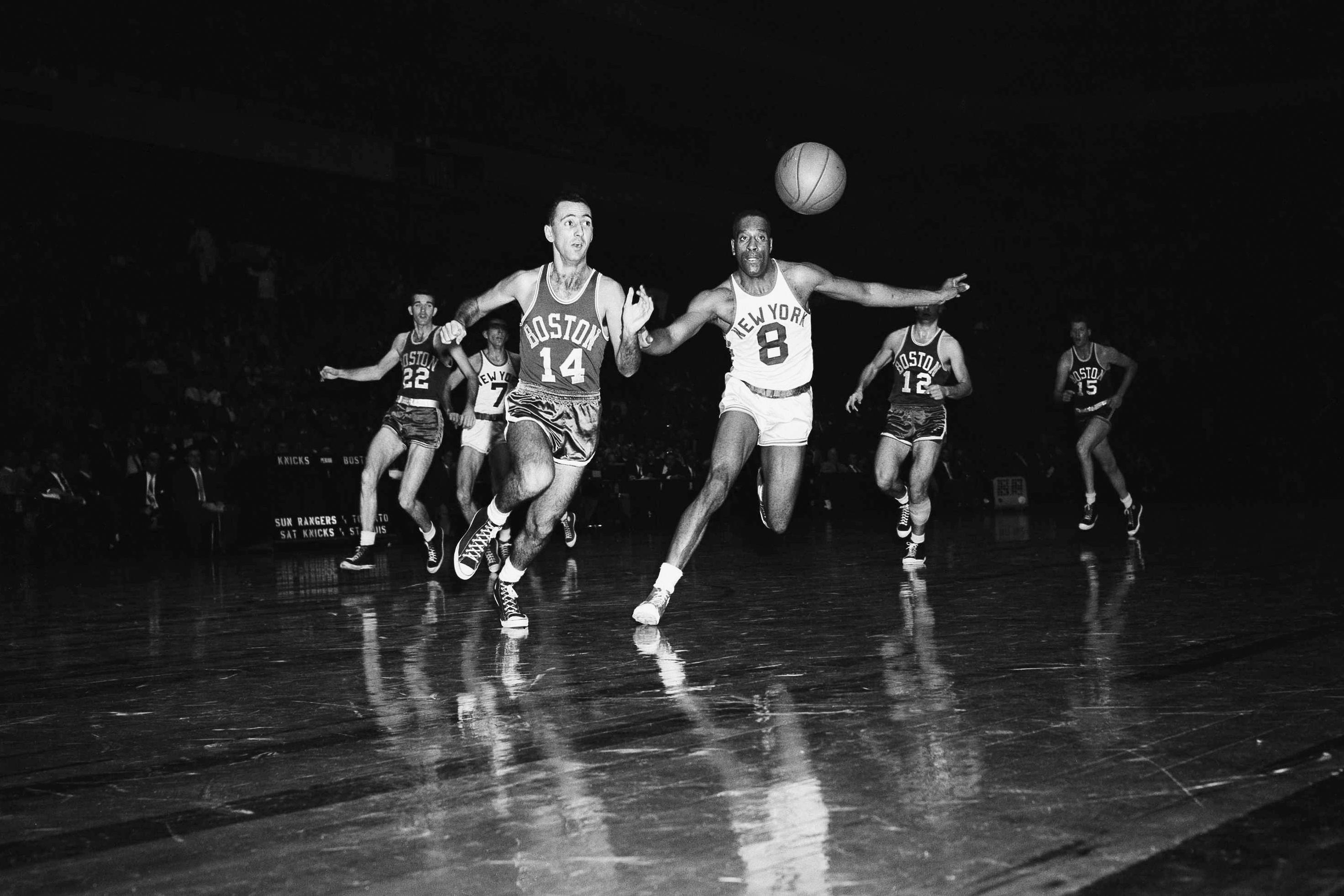In this darkly lit image, a basketball game unfolds on a shiny, reflective wooden court featuring players from the Boston and New York teams. Four Boston players in darker jerseys and shiny satin shorts—numbered 14, 12, 15, and 22—dominate the scene along with two New York players in white jerseys—numbered 8 and 7. The players are captured in intense action, sprinting and vying for a loose ball, their muscular forms emphasizing the athleticism of the moment. Despite the bright lights necessary for the game, the background fades to black, obscuring details of the bench and spectators, creating a dramatic focus on the players and their high-energy chase.